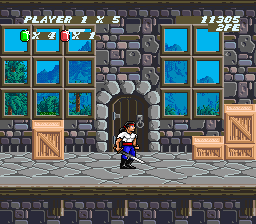This image is a detailed snapshot from an older side-scrolling video game, depicting a scene with a pixelated character standing on a cobblestone roadway. The character, a somewhat muscular male, is adorned in a white shirt, blue pants, black boots, a red belt, and a red bandana tied over long black hair. He wields a sword in his right hand, featuring a gold handle and a steel-gray blade, pointing to the right. Behind him stands a stone castle wall with a large wooden door at its center, flanked by multiple square windows through which a mountainous valley and some trees are visible. Wooden crates are stacked on both sides of the walkway, contributing to the medieval and adventurous atmosphere of the game. Additionally, a heads-up display at the top of the screen provides game status information such as "Player 1 x 5 green jewels times 4 red jewels times 1:1:3:0:5:2 FE."